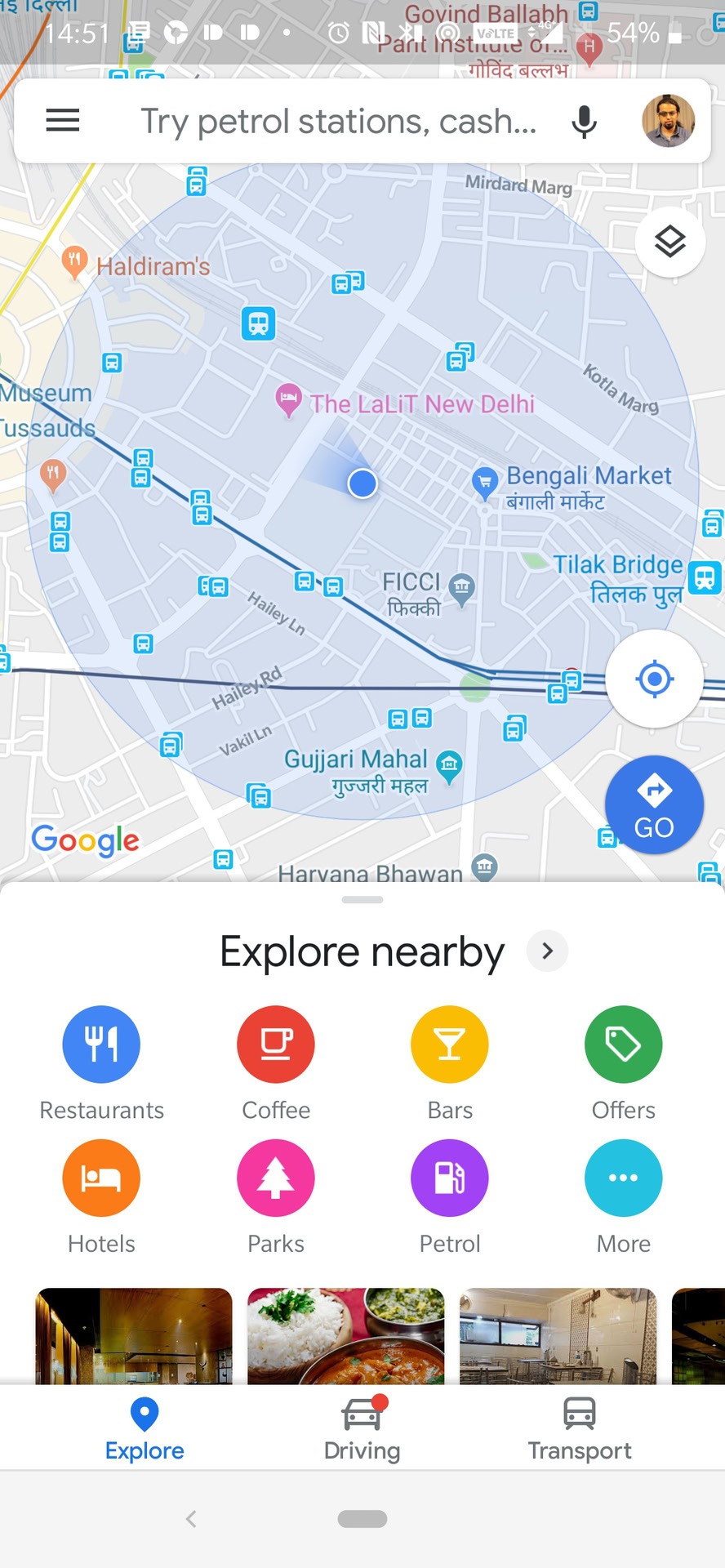This is a detailed screenshot of a map application displayed on a mobile phone. The top section features a translucent gray header displaying '1451' in white on the left side, accompanied by a row of various icons positioned to the right. Directly beneath the header is a white search bar with three horizontally stacked black lines on the left side, grey text stating "try petrol stations, cash,..." in the center, followed by a black microphone icon and a circular profile picture of a man on the right.

The main portion of the screenshot highlights the map itself, characterized predominantly by white street lines. Several transit lines are apparent, with one running horizontally across the map and another angling upward to the left at a 45-degree angle. Scattered along these lines are bright blue bus stop icons featuring white bus symbols, as well as additional bus stop icons located on larger roads.

The map is labeled with a mixture of English and Hindi names and dotted with various geolocation pins in orange and pink. A prominent pink pin is situated in the center, marked by text reading "The Lalit New Delhi."

Additional map interface elements include a white circle with two vertically stacked dark gray diamonds located beneath the search bar on the upper right, and two circles at the bottom right corner. The top circle is white with a blue reticle icon in its center, while the circle below it is blue, inscribed with white text at the bottom that reads "GO" and a white diamond with a blue right-pointing arrow above.